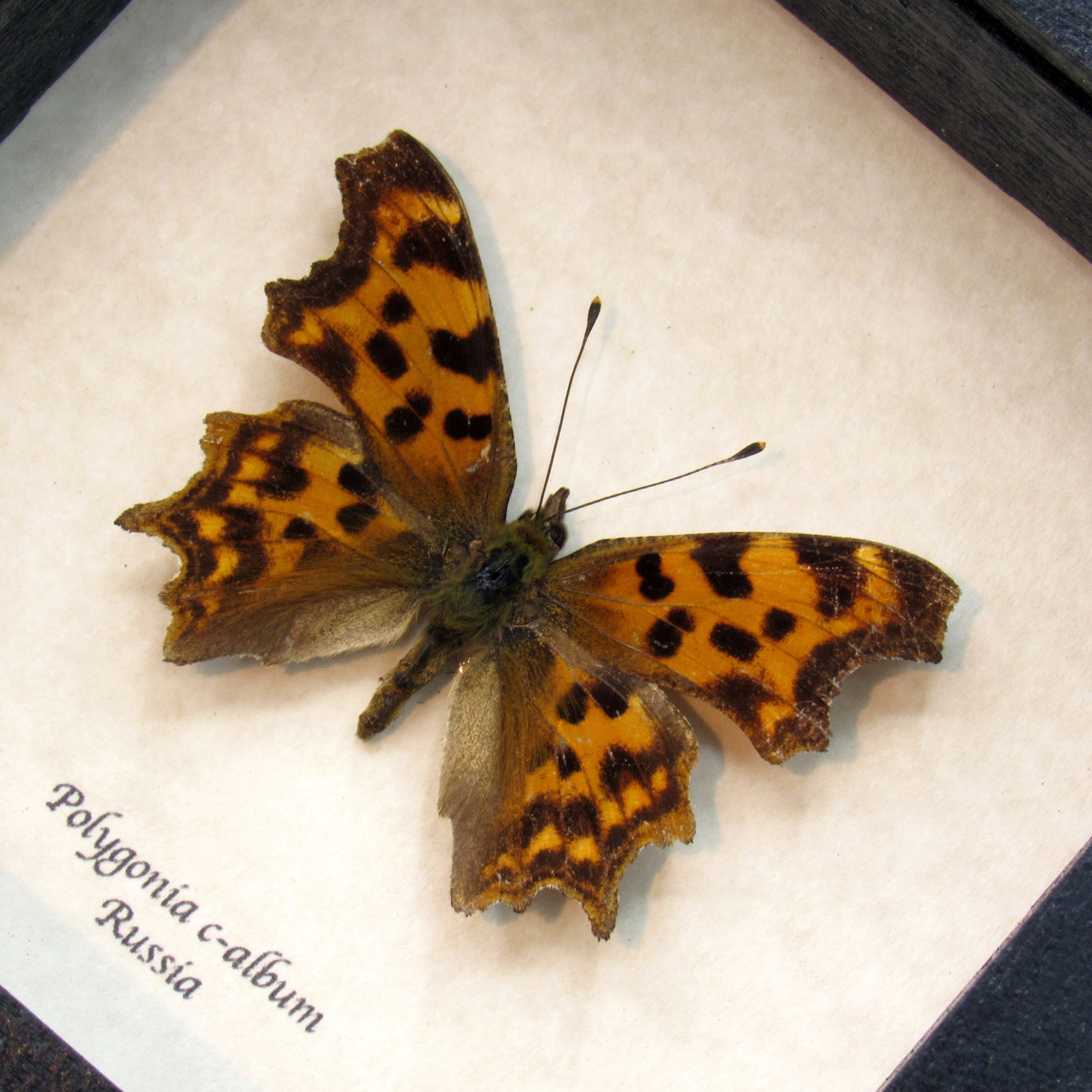This photograph captures a preserved butterfly, identified as Polygonia C album, originating from Russia, centered within a wooden-framed glass case. The butterfly, positioned slightly tilted to the right, rests on white paper that covers most of the background. The intricate details of its wings showcase a predominant orange hue with black and brown spots, particularly on the lower wings, and tan-yellow highlights. The butterfly's body is vertically aligned, with the bottom right wing extending down and the top left wing spread open wide. Its long antennas extend from its sizable, brownish body. The text "Polygonia C album Russia" is noted in the bottom left corner of the paper, emphasizing its scientific classification and origin. The case's frame, with its blackish-blue tint, forms a subtle border at the top right, top left, bottom right, and bottom left corners. Overall, the display exudes a scientific and elegant presentation, highlighting the beauty of this preserved Russian butterfly.